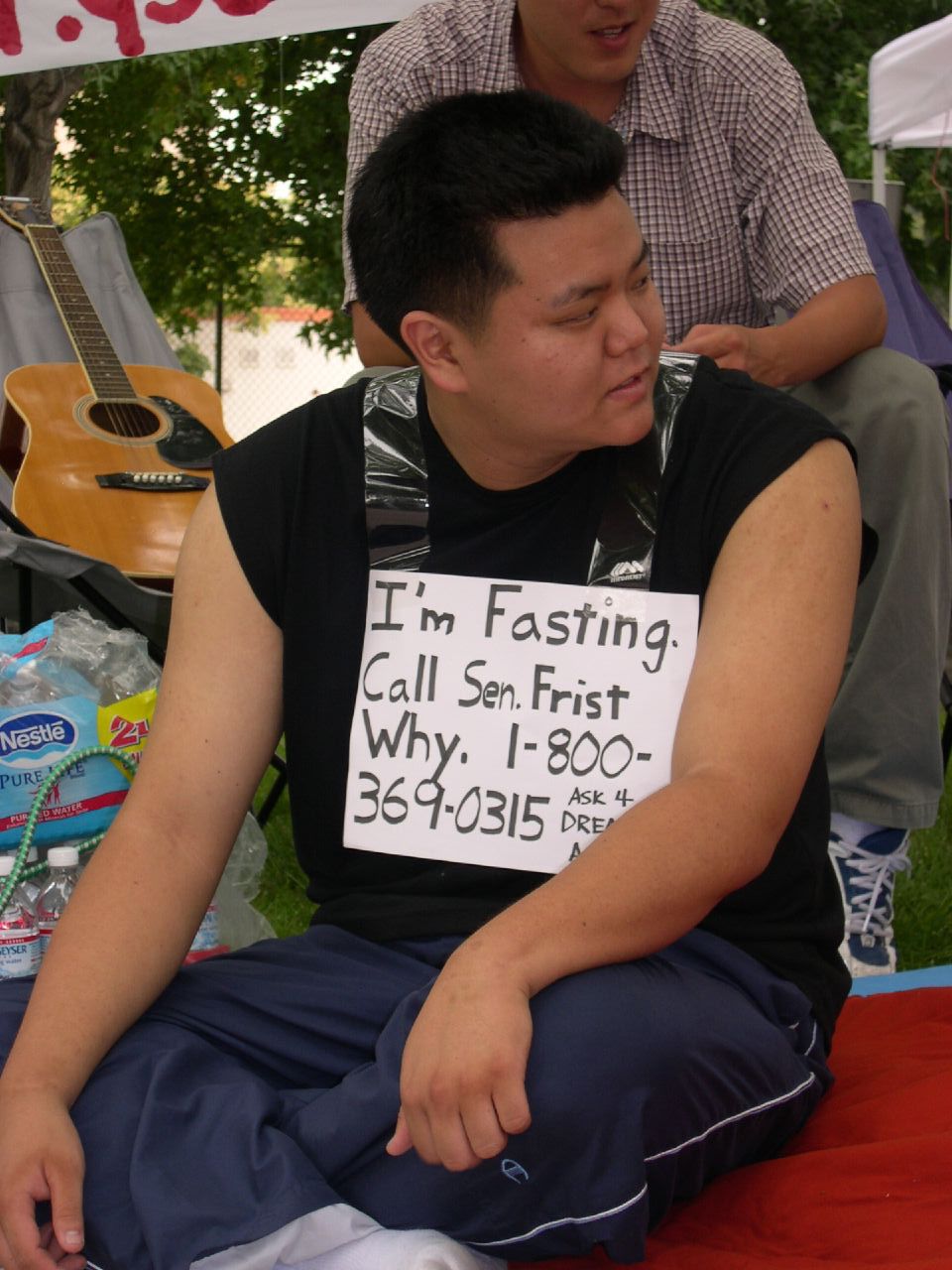The image captures an outdoor scene featuring a young Asian man with short dark hair, sitting cross-legged on a red blanket. He is wearing a black tank top and blue Champion wind pants with a distinctive white stripe down the leg. Around his neck is a white paper sign attached with plastic straps, partially obscured by his arm. The sign, written in bold Sharpie, reads: "I'm fasting, call Senator Frist, Y 1-800-369-0315." Positioned behind him are 24-pack cases of Nestle Pure Life bottled water and an acoustic guitar. Further back, a man can be seen wearing a button-up shirt, khaki pants, and white and blue tennis shoes. The backdrop includes a tree with abundant leaves and a fence, highlighted by natural outdoor lighting. Additional details include red lettering on a white banner in the top right corner of the photo, adding to the vibrant scene.